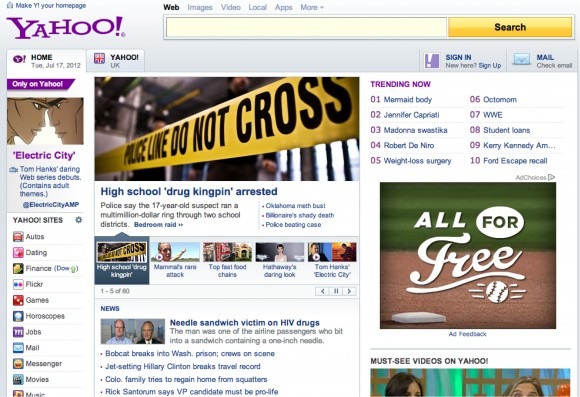This image is a screenshot of the Yahoo home page from Tuesday, July 17th, 2012. The design and format are distinctively different from contemporary layouts, marked by a nostalgic, somewhat cartoonish look. The old Yahoo logo is prominently displayed in the upper left-hand corner, featuring "Yahoo" written in jovial, purple letters against a subtle, very light lavender background.

Near the top left, the date is clearly visible. Below the logo, a gold-colored, rectangular search button with "Search" inscribed in white is positioned beside a long, white search box. The "Trending Now" section, listed in purple, offers a peek into July 2012's popular topics, including "Mermaid Body," "Jennifer Capriani," "Madonna Swastika," "Robert De Niro," "Weight Loss Surgery," "Octomom," "WWE," "Student Loans," "Carrie Kennedy," and "Ford Escape Recall," though some trends remain cut off in the screenshot.

Dominating the center top is a large photograph of a yellow police line, which typically appears at crime scenes. The words "Police Line Do Not Cross" are clearly printed in black font on the tape. The corresponding headline, written in blue and prominently positioned, reads "High School Drug Kingpin Arrested."

On the right side, just below the trending topics, there's a visually engaging ad. This square advertisement is divided into two halves: a dark green upper section and a brown lower section, reminiscent of a ball diamond. Written in white, the ad enticingly states "All for Free," accompanied by a drawing of a white baseball, capturing attention with its simplistic yet effective design.